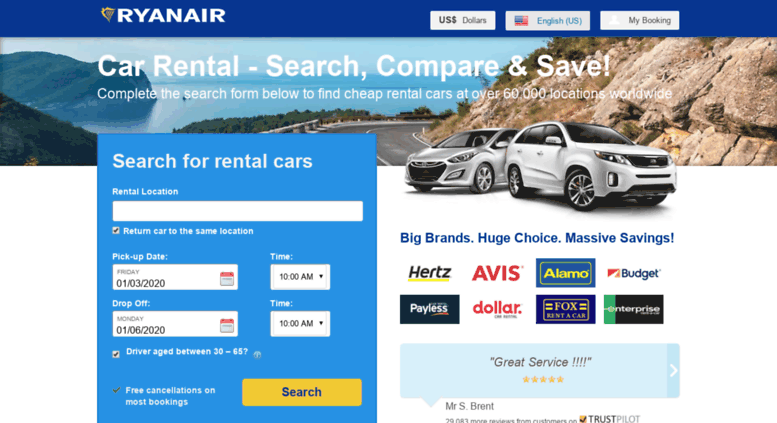The image features a rental car search webpage, prominently displaying the text "Car rental, search, compare, and save." Users are prompted to "complete the search form below to find cheap rental cars at over 60,000 locations worldwide." The form fields include an empty text box for specifying the rental location, with instructions to search for rental cars. The background showcases scenic imagery, featuring two cars— a sedan and an SUV— parked on a road. The road is situated on a hill with picturesque mountains in the distance. The pickup date is set for January 3rd, 2020, and the drop-off date is January 6th, 2020. The color palette of the scene includes shades of blue, yellow, white, silver, brown, and green.